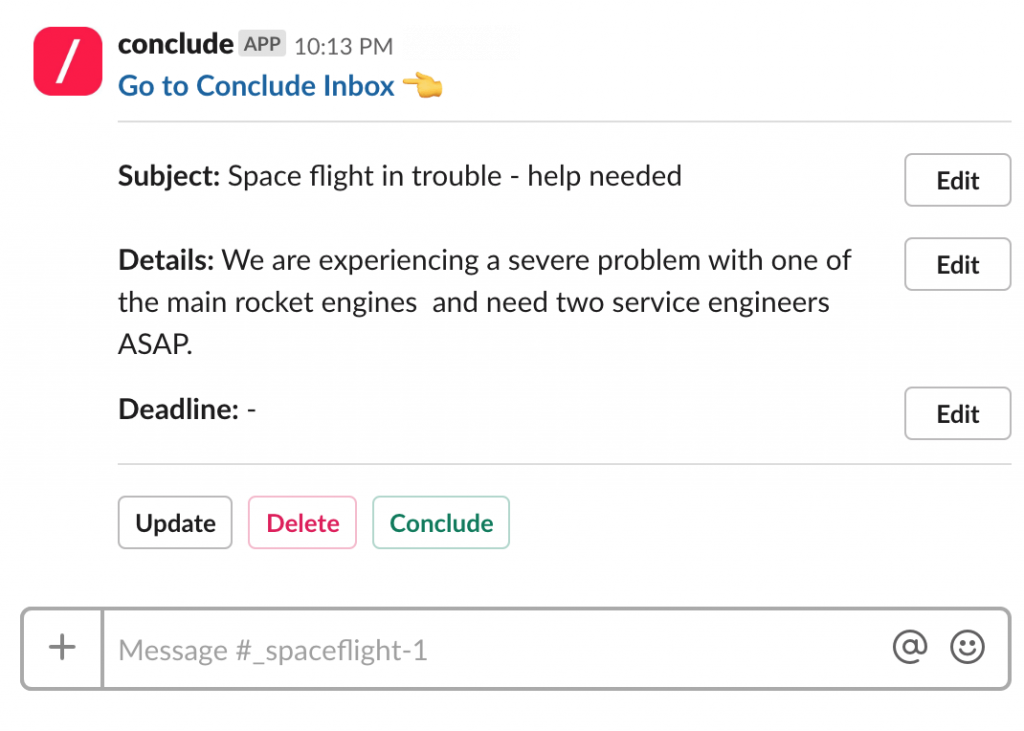The webpage features a clean white background. In the upper left-hand corner, a prominent red box catches the eye, featuring a white dash horizontally aligned through its center. Adjacent to this red box, the word "Conclude" is boldly displayed in black font. Nearby, a small gray box contains the text "APP" also in gray, followed by "10.13 PM" in similar styling. Below these elements, a directional prompt in blue reads "Go to Conclude Inbox," accentuated by a yellow hand icon pointing towards it.

A gray horizontal line stretches across the page, demarcating sections. Below this line, a key subject heading appears as "subject.spaceflightintrouble-helpneeded." Directly to its right, a black-outlined rectangle featuring the word "edit" offers interactive functionality.

The subsequent section labeled "details" communicates a critical message in black text: "We are experiencing a severe problem with one of the main rocket engines and need Two Service Engineers ASAP." The urgency is highlighted by capitalizing "ASAP." Another gray "edit" box is positioned here for content modifications.

Below this detail, another section titled "deadline" is accompanied by an additional "edit" button in a similar gray-outlined box. Another horizontal gray line extends across the page, providing further separation.

The interface concludes with three interactive boxes at the bottom: one outlined in gray with the word "update" in black, another outlined in red with "delete" in red, and the last one outlined in green featuring the word "conclude" in green. A longer gray box at the bottom of the page includes the message "message_hashtag_spaceflight-1," framed by the additional underscore and hyphen characters for emphasis.